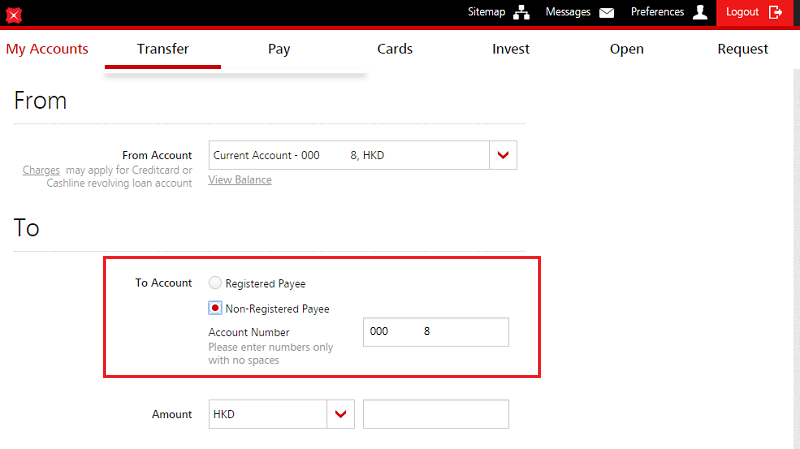The image is a detailed screenshot of a banking application interface on a computer screen. In the top left corner, a red square with a white 'X' is visible. On the top right, navigation options read: "Site Map," "Messages," "Preferences," and "Logout." 

Below these options, a horizontal navigation bar displays labeled sections: "My Accounts" in red, "Transfer" with a red underline, "Pay," "Cards," "Invest," "Open," and "Request." 

In a larger font underneath, the screen prompts "From," followed by "From Account" and a note stating, "Charges may apply for Credit Card or Cash Line Revolving Loan Account." A text box labeled "Current Account 0008HKD" with a "View Balance" hyperlink is also present.

Moving down, the prompt "To" appears, accompanied by a red-bordered rectangle labeled "To Account." Below, two options are presented: a circle to select "Registered Payee" (unfilled), and another circle filled with red, within a blue box, indicating "Non-Registered Payee."

Further down, instructions state, "Account Number. Please enter numbers only with no spaces." A text box adjacent to this has partially filled numbers: "000, _____, 8."

Lastly, an "Amount" field features a drop-down box pre-filled with "HKD," accompanied by a downward-facing arrow. To the right of this box is another text box, currently void of any text.